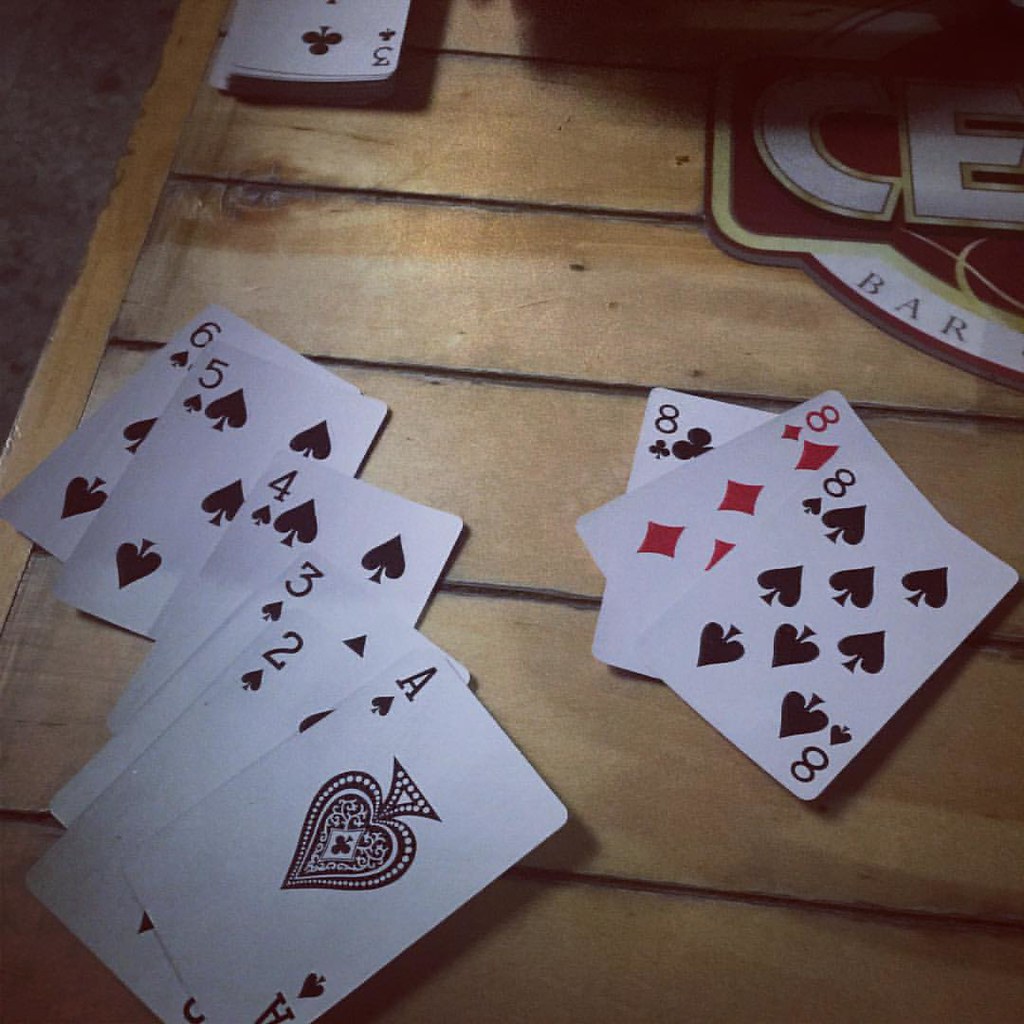The photograph depicts a wooden surface, which might be a table or possibly a floor. Scattered across this wooden surface are various playing cards. In the upper left corner of the frame, part of a dark brown shaggy carpet is visible. Near this carpet, and slightly off the left-hand side of the image, is the lower half of a deck of cards, with the revealed top card being a three of clubs.

In the lower left-hand corner of the photograph, six sequential cards are neatly arranged: the ace, two, three, four, five, and six of spades. Notably, the four of spades appears to be slightly bent. 

On the right-hand side of the image, a little above the bottom edge, there are three cards displayed: the eight of clubs, eight of diamonds, and eight of spades. Positioned above these cards is a red coaster with gold and white detailing. The coaster is partially obscured by a shadow, but it reveals the letters "CE" and the word "bar" in black text on a white band at the bottom.